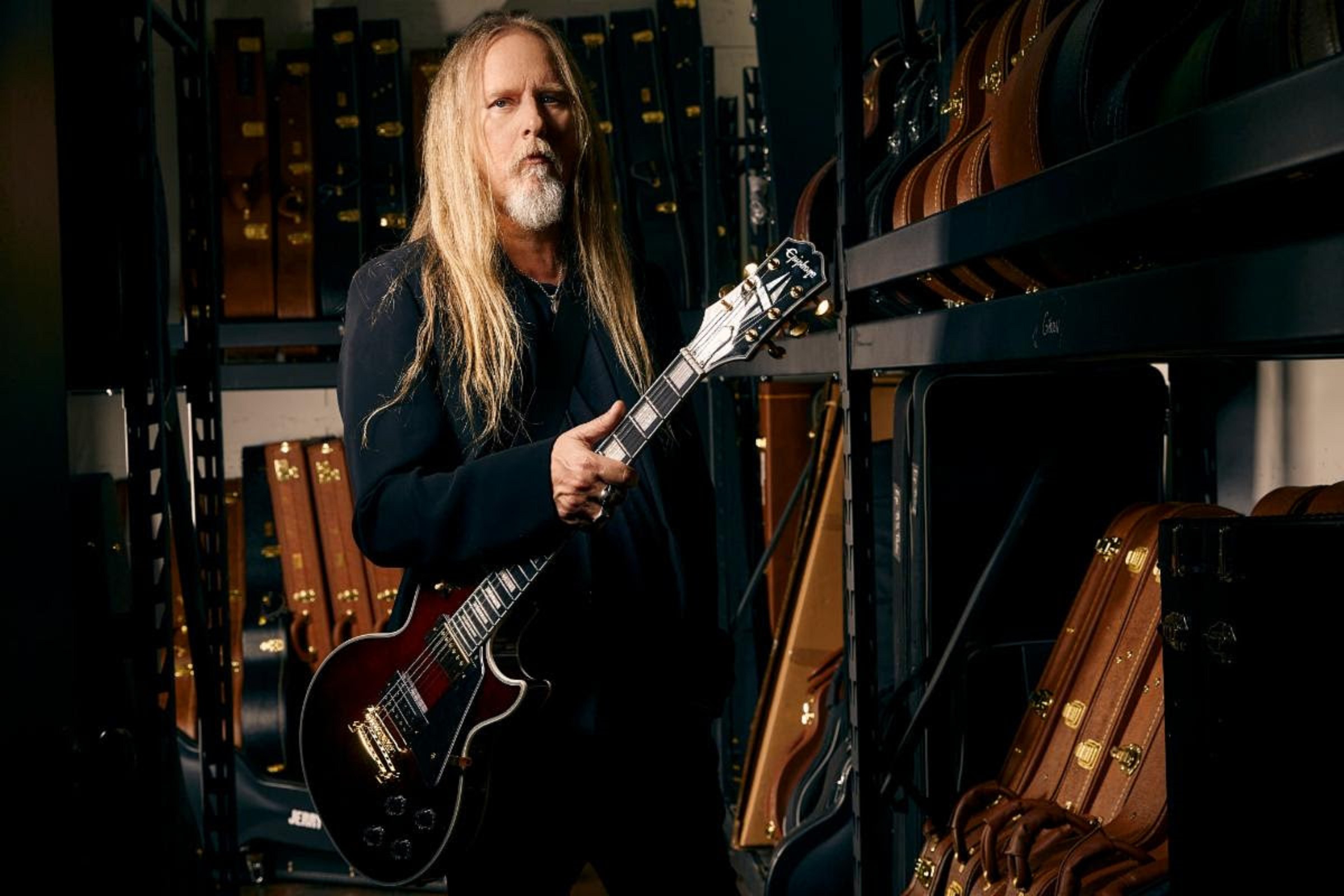This detailed color photograph captures Jerry Cantrell, the renowned rock musician famously known for his role in Alice in Chains during the early to mid '90s. He stands in a room filled with approximately 20 tan and black leather guitar cases, each secured with brass buckles, neatly arranged on black metal shelves. Jerry, with his long, straight blonde hair and distinctive white goatee, commands the viewer's attention with an intense, serious gaze. He's dressed in a black suit jacket and dark pants, accessorized with a silver cross necklace. In his hands, he cradles a dark cherry red Epiphone electric guitar, adorned with shiny gold hardware, highlighting his rock star persona amidst the dimly lit, moody atmosphere of the room.